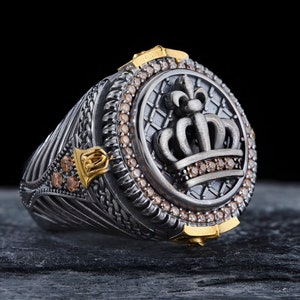This photograph captures a substantial, opulent men's ring that appears to be crafted from pewter with striking gold accents. The centerpiece of the ring is a round face, prominently featuring a crown encircled by several layers of intricate design. The outermost layer showcases small metal spines or ridges, while the next layer is adorned with round, brown stones that add a touch of richness. Beneath the crown, there are five more stones that resemble diamonds, though their brilliance is understated due to the angle and lighting of the shot.

The band of the ring is equally detailed; it boasts gold etchings and chevrons, as well as unique elements like a triangular arrangement of slightly larger brown stones on the side, pointing downward. The ring also has gold brackets connecting the face to the band, enhancing its elaborate and antique aesthetic. Though the precise materials are difficult to pinpoint from the photograph, the ring exudes an aura of heavy, regal elegance, suggesting it may be a vintage or heirloom piece.